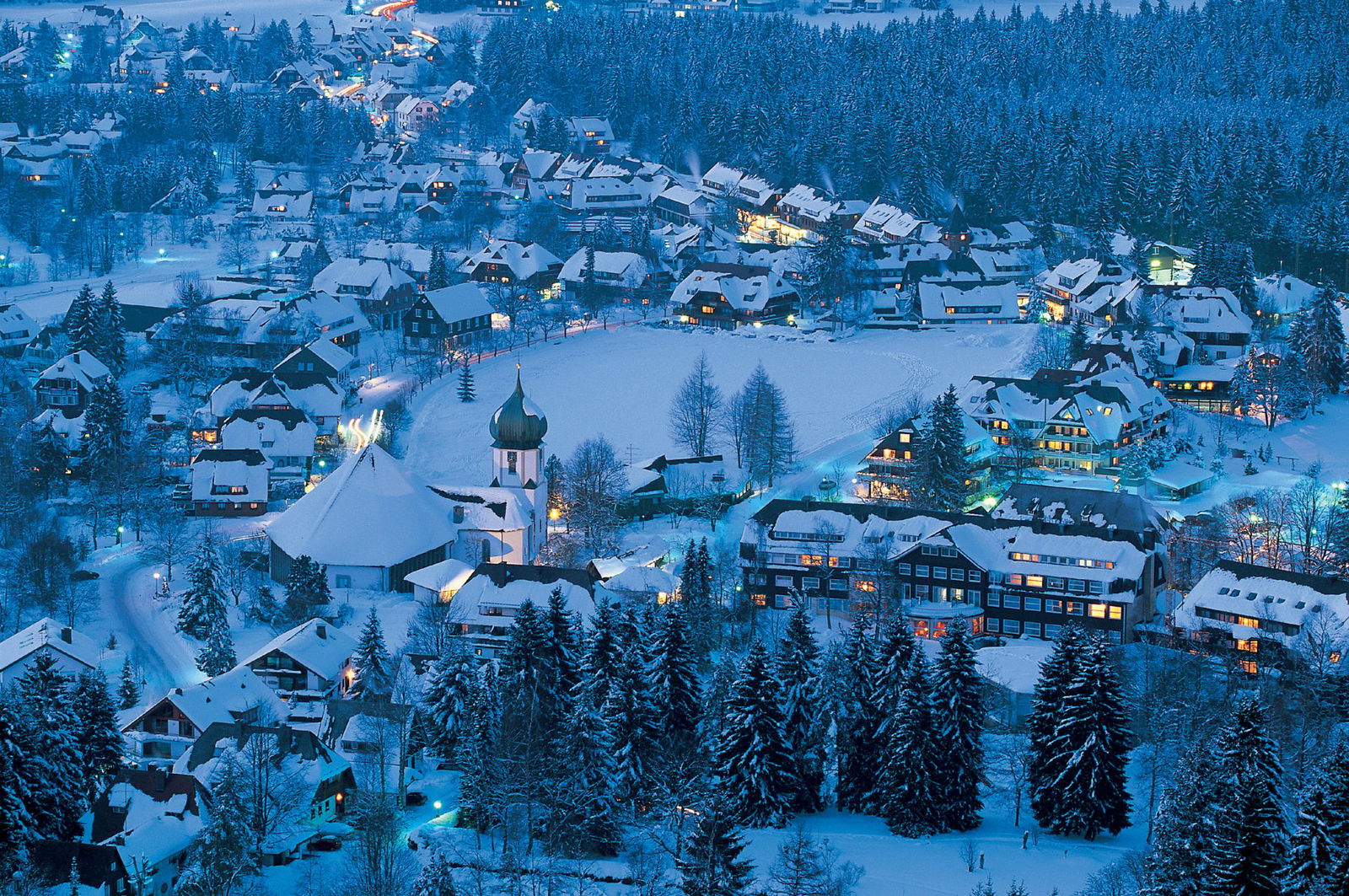An aerial photograph of a quaint village, possibly a ski resort or a cold winter retreat, captured during the enchanting blue hour—just before sunrise or shortly after sunset. The scene is bathed in a serene bluish hue, enhancing the picturesque winter landscape. The village comprises predominantly two-story wooden buildings, their warm lights glowing softly in the early morning gloom. Dominating the skyline is a taller structure, likely an Orthodox church, its distinctive dome rising gracefully above the rooftops. The snowy backdrop is adorned with dense forests, adding to the tranquil beauty of the setting. At the heart of the image lies a frozen, snow-covered lake, seamlessly blending into the wintry panorama.